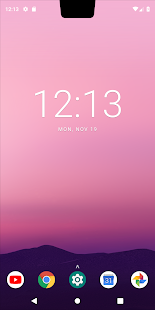This image captures the home screen of a smartphone featuring a visually appealing gradient wallpaper. The top of the wallpaper starts with a light pink hue, transitioning smoothly into darker shades as it moves downward. Toward the lower part of the screen, subtle cloud-like colors appear, blending into a serene landscape of rolling purple mountain ridges. The bottom 20% of the screen is a solid color, housing five prominent menu icons: YouTube, Chrome, Settings, Calendar (showing the date as the 31st), and the Google pinwheel icon.

Below the icons is a navigation bar. In the upper left-hand corner of the screen, the time is displayed as 12:13, with a few indistinct icons to the right of it. The upper right-hand corner shows the Wi-Fi signal strength and battery status. The top center of the screen features a cutout with angled sides, which is the black chin space for the camera. At the center of the screen, large white bold text displays the time "12:13," with "Monday, November 19th" written beneath it.